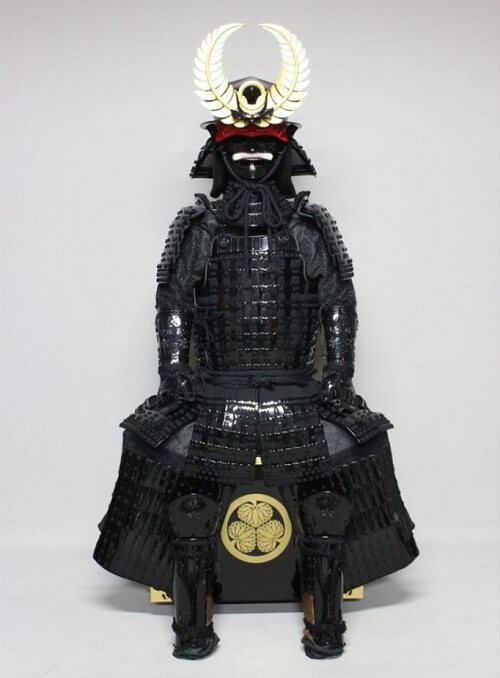This image depicts a highly detailed, lifelike, computer-generated representation of a sitting figurine or person adorned in elaborate, black, shiny vinyl or metallic armor that resembles a blend of a superhero outfit and traditional Japanese warrior garb, possibly samurai. The armor is comprehensive and covers the entire body, including glossy black boots and gloves. The helmet features striking white feather-like structures that curve and resemble horns, adding to its dramatic appearance. The facial area is shielded with a black mask that has a subtle white opening for the eyes. The figure is seated on a black stool. Notably, between the figure’s legs, there is a distinctive golden circle adorned with three spade-shaped leaves or pumpkin-like shapes, enhancing the intricate and regal appearance of the ensemble.